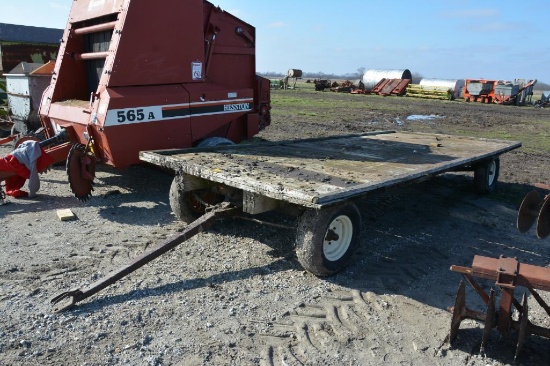This color photograph in landscape orientation captures a detailed scene of a commercial agricultural site on a clear, sunny day with a bright blue sky. Dominating the center, there is a flatbed wagon designed for hauling, equipped with black tires featuring white hubcaps. The flatbed, which has a simple wooden surface without any railings or compartments, lies slightly angled with its metal chain hitch extending forward toward the lower left corner of the image. The wagon rests on a dusty dirt road strewn with gravel, showcasing visible tire tracks.

To the left of the wagon, a red mechanical object with a white trim and a chute at the front catches the eye. This piece of machinery, also partly obscured but seemingly designed for processing or compacting materials, has a thick, hitch-like boom extending forward, similar to the flatbed wagon. Further to the right is another unidentifiable metal mechanical apparatus, adding to the array of equipment depicted in the field.

In the background, a wide, muddy field stretches out to the horizon, dotted with additional agricultural equipment. Beyond the field, there are large, warehouse-like structures, possibly aluminum, resembling storage hangars for harvested crops. The clear demarcation of these elements against the vibrant sky gives a sense of the expansive, industrious setting of this agricultural landscape.